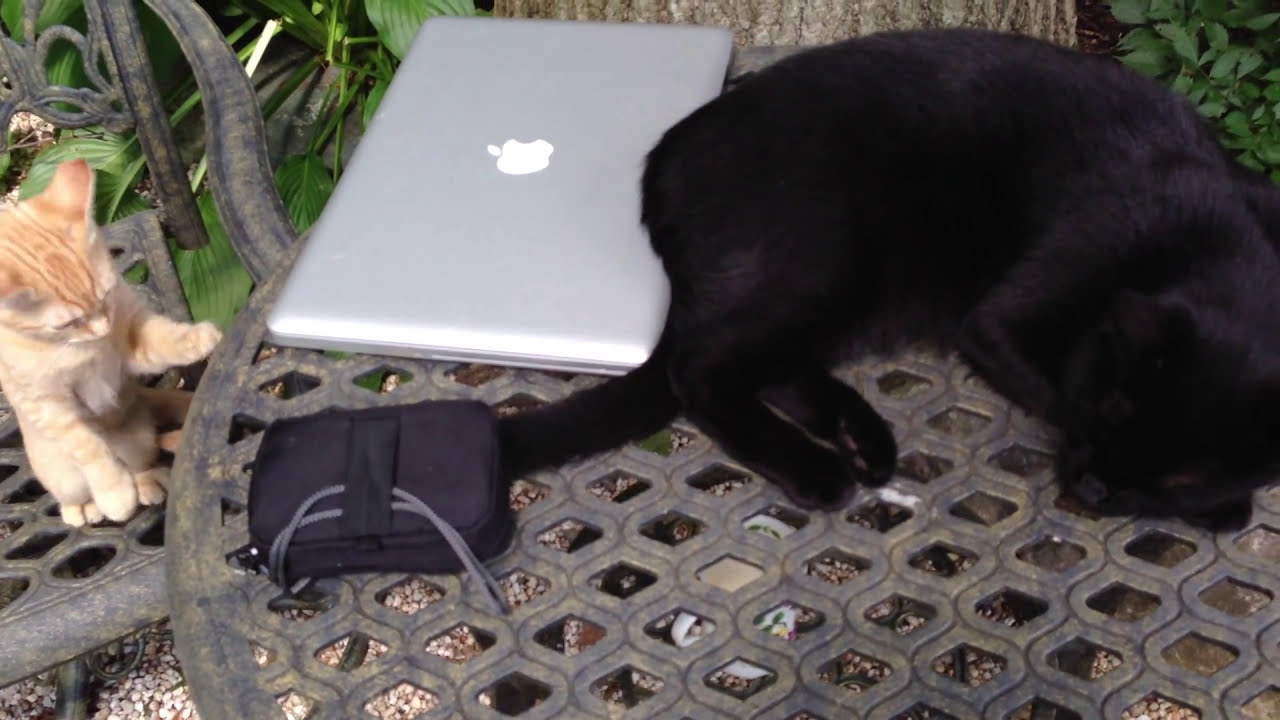This full-color, horizontal photograph captures an outdoor scene featuring two cats amidst a tranquil setting. In the foreground, a black adult cat is curled up and asleep on a round, metal table with a grated surface. Positioned on the left side of the frame, a curious brown-orange kitten stands on its hind legs, one paw reaching up to the table from a matching metal chair. The table also holds a silver Apple laptop, identifiable by the iconic white logo on its lid, placed behind the black cat. Additionally, a black phone case lies near the edge of the table. Surrounding the scene, the trunk of a tree and lush green leaves from various plants add to the picturesque, daytime ambiance.